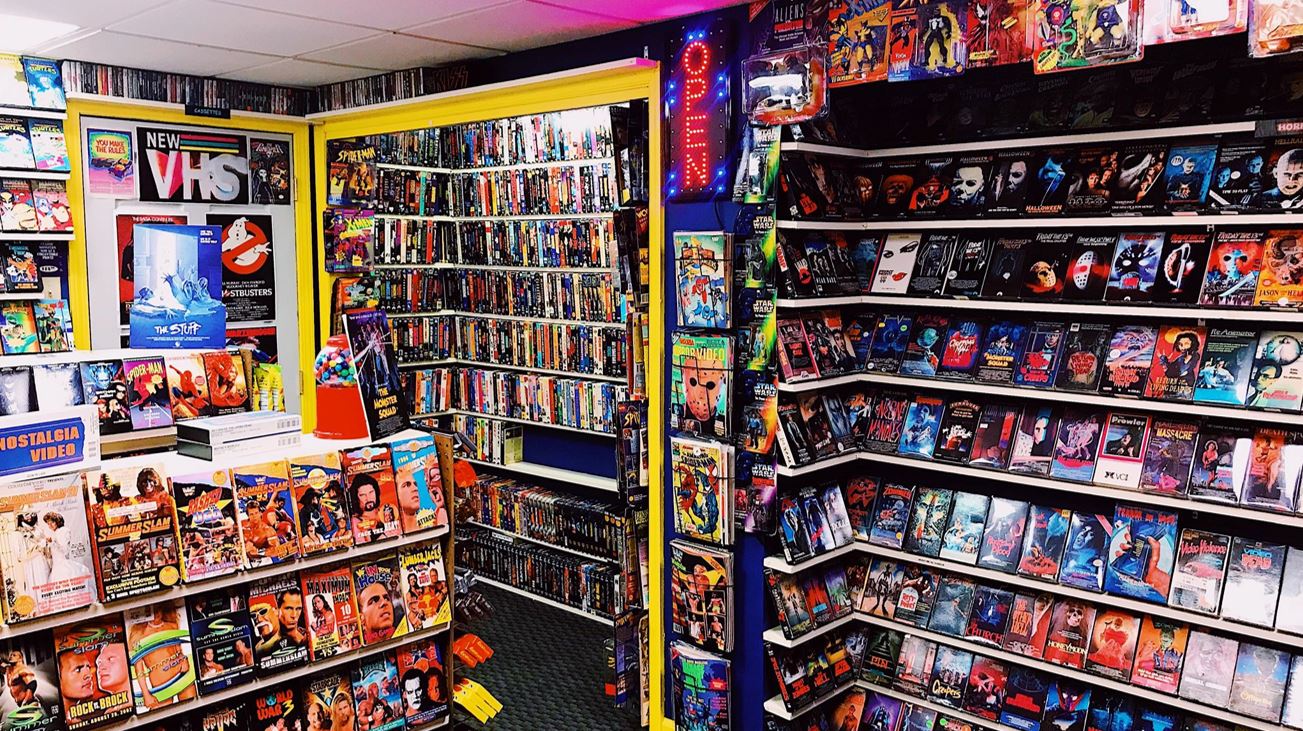This color photograph in landscape orientation captures the interior of an old-school video rental store, reminiscent of the days when VHS tapes were the primary medium for home entertainment. The store, identified as "Nostalgia Video" by a sign in the top left corner, is brightly lit and exhibits clear image quality. Prominently featured on the right side is the horror section, with rows of VHS tapes including iconic titles such as "Friday the 13th," "The Prowler," "Texas Chainsaw Massacre," and "Honeymoon." The center of the store contains additional shelves stocked with various videos, as well as some comics. A standout feature is a neon sign in the top center reading "OPEN" in red letters, accented by blue lights. To the left, another area displays even more VHS tapes, along with a counter that has a few VHS videos on it and a rack in front. The overall layout of the store includes various niche areas painted in yellow, filled with a wide array of VHS cassettes that stretch across the entire space. The realism of the photograph vividly evokes the nostalgic ambiance of a bygone era of video rental.